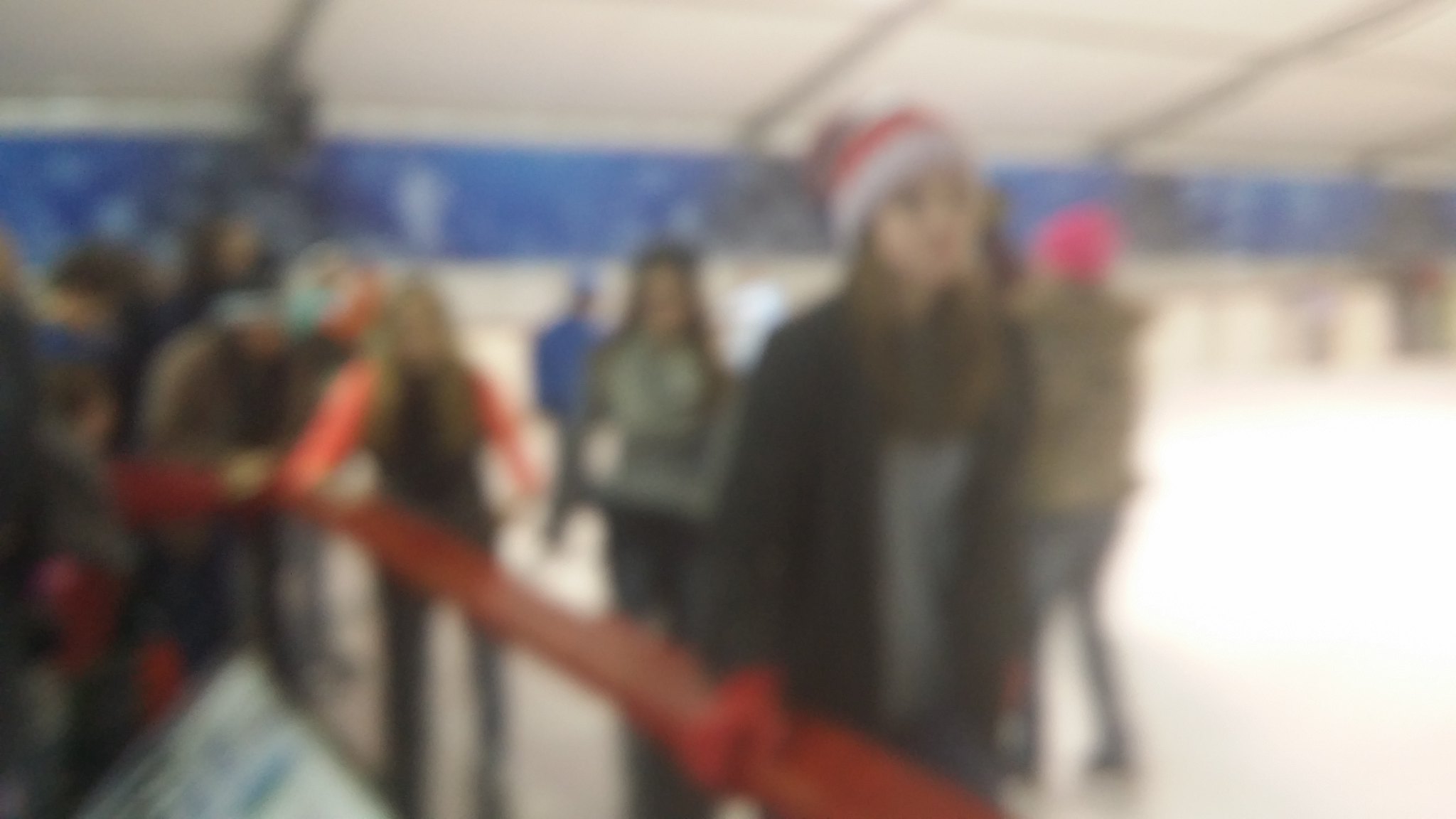This is a very blurry photograph capturing a group of people ice skating. The scene is set in an ice rink, which is dominantly white with a slightly arched white roof. The background features a dark blue wall with white markings or lines. The foreground highlights an orange-red handrail, secured to the floor by black poles, which the skaters use for support.

Among the group, the most visible person is a young woman with long brown hair. She is dressed in a black jacket over a gray t-shirt, wearing red gloves, and a red and white Santa Claus hat. Nearby, another skater can be identified by their bright pink beanie. A woman behind the central figure has long blonde hair, an orange-sleeved shirt, and what appears to be a black vest. Several other skaters with long hair also populate the scene, adding to the lively yet blurred activity in the rink.